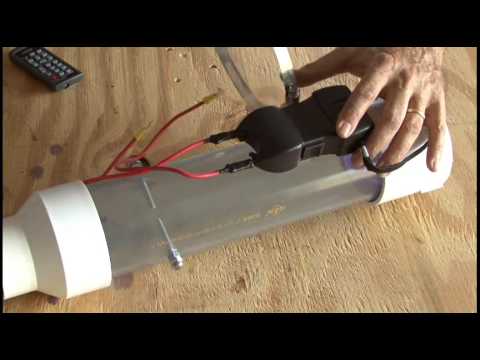A detailed photograph captures a close-up scene set on a light brown plywood surface, marred with various dents and breaks. Dominating the center of the image is a clear cylindrical tube, likened to the type used at bank drive-throughs, with white plastic caps on both ends. Resting on this tube is a black object resembling a taser, identifiable by its long black points from which red wires emerge. These wires extend to the left, then curl back towards the right in a delicate arc. A white person's hand enters the frame from the upper right corner, fingers open and thumb spread. Adorned with a thin golden ring on the ring finger, the hand delicately grips the black object, with the fingers just touching its sides. Nearby, in the upper left corner of the image, a black remote control with gray buttons is visible. Additionally, next to the black object, a clear item with a silver frame stands on its side, possibly a magnifying glass. The photograph itself is bordered by thin black edges on the sides and slightly thicker black borders on the top and bottom.